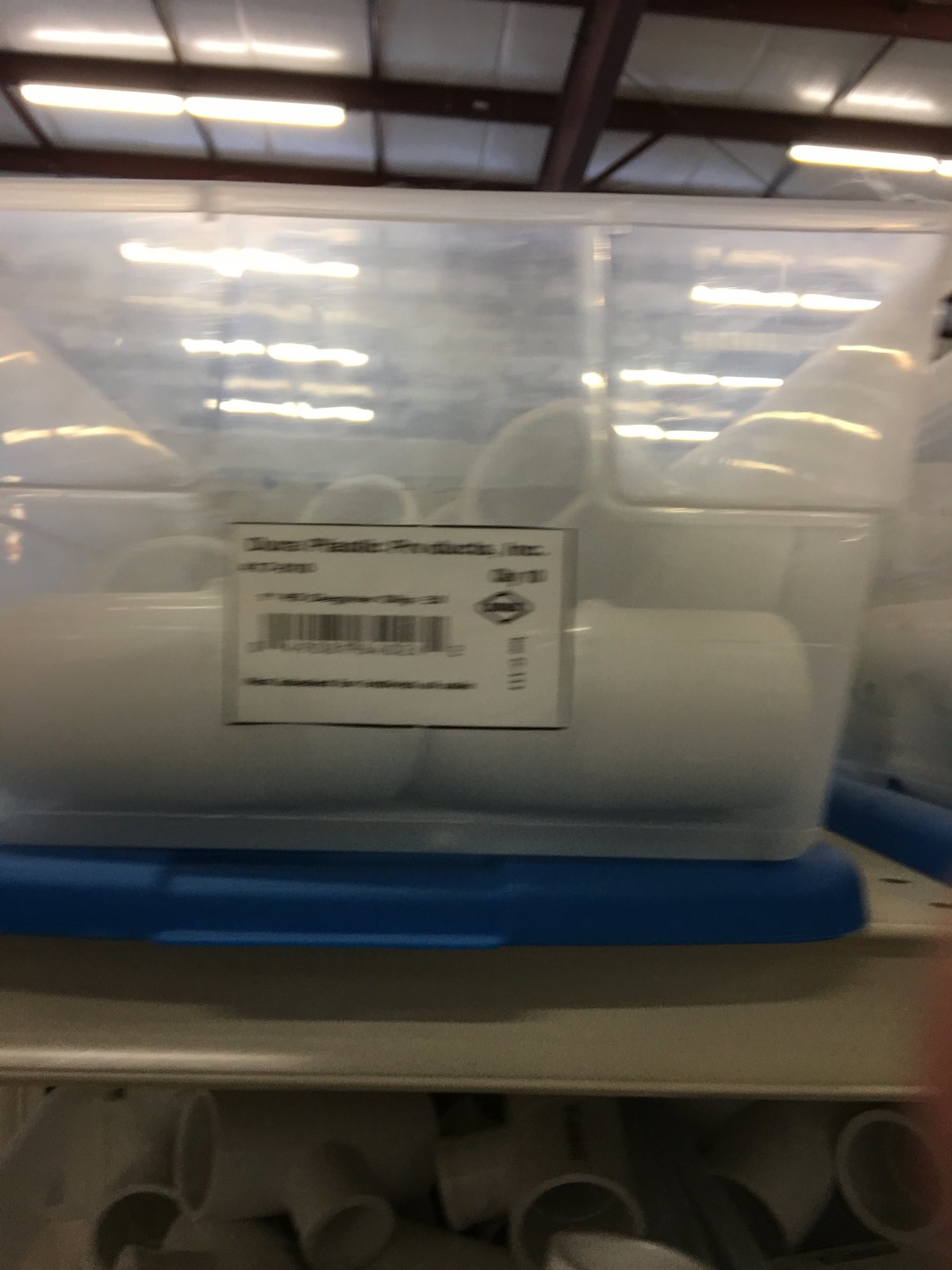This photograph captures the interior of a retail store, focusing on a cream-colored metal shelving unit. On the top shelf, there is a clear plastic rectangular bin, which is resting on a royal blue lid. Inside this bin, there are several short pieces of white PVC pipe. The front of the bin features a white label, which appears to detail information about the PVC products, although the text is too blurry to decipher clearly. On the lower shelf, additional short pieces of white PVC pipe are visible, though the exact nature of their storage is concealed from view. This image highlights an organized yet utilitarian display within a hardware or home improvement store setting.